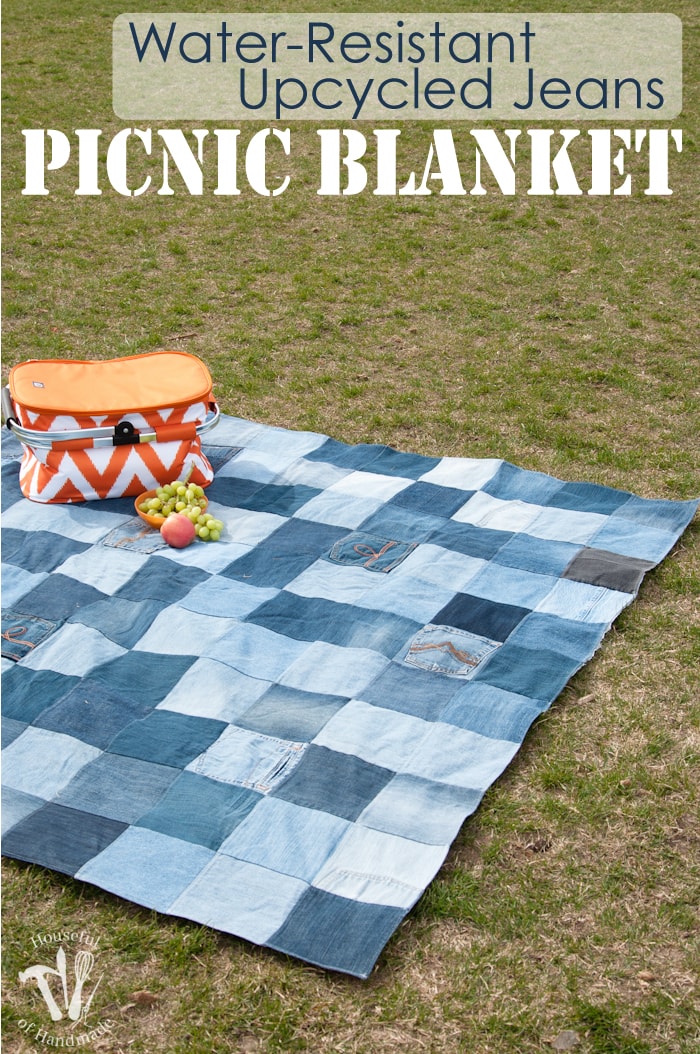The photograph depicts a picnic scene set on a flat, grassy area that includes clumps of dirt and patches of dead grass. Centrally featured is a picnic blanket made from small squares of blue denim, showcasing various shades and back pockets from upcycled jeans. This unique blanket is marked with stenciled white letters reading "Picnic Blanket" directly below a semi-transparent white rectangle with blue text stating "Water Resistant Upcycled Jeans." The bottom left corner of the image displays a logo for "Houseful of Head Maid," accompanied by graphics of a hammer, pick, whisk, and fork in white text. 

Arranged on the stylish denim blanket is a prominent orange and white striped picnic basket with silver handles, as well as a bowl brimming with fresh green grapes. An eye-catching detail includes the picnic basket's chevron-patterned sides. An additional detail of the scene includes a small red apple placed on the blanket near the bowl of grapes, enhancing the inviting, rustic appeal of the picnic setup.